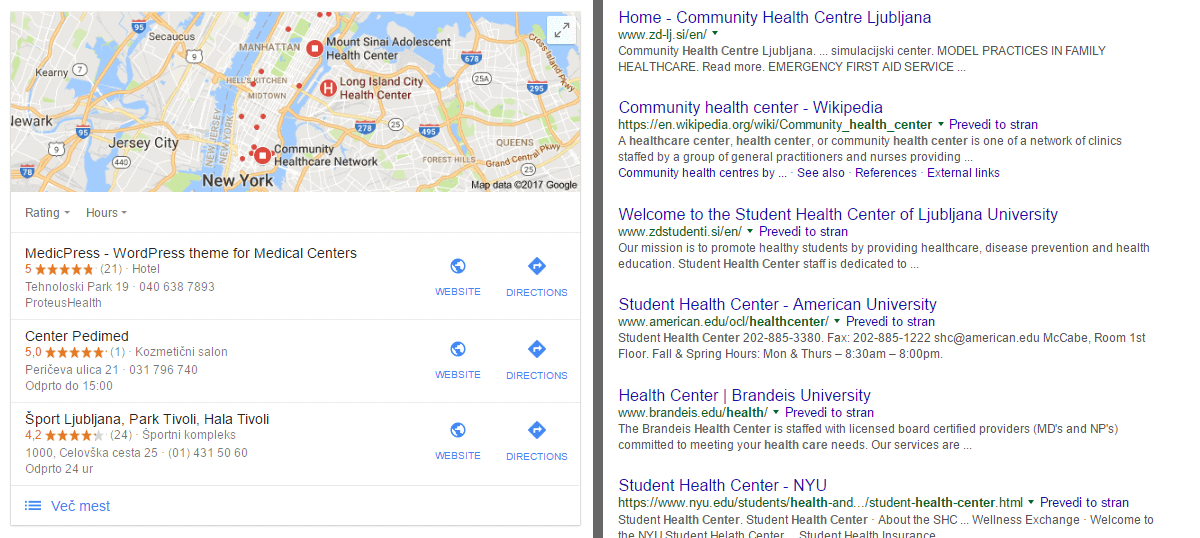The image comprises two detailed screenshots side by side. 

On the left side, there is a Google Maps screenshot featuring a section near New York City, particularly focusing on Manhattan. Below the map are three links related to locations marked on the map:
1. **MedicPress** - A WordPress theme for medical centers with a five-star rating. Accompanied by website and directions icons.
2. **Center Paramed** - Also rated five stars and accompanied by website and directions icons.
3. **Sport, Ljubljana, Park, Tivoli, Hala Tivoli** - This listing also includes website and directions icons.

The right half shows a "Results and Research" page, listing six websites from top to bottom:
1. **Community Health Center Ljubljana** - With its URL and a brief description.
2. **Community Health Center Wikipedia** - Followed by its URL and a brief description.
3. **Welcome to the Student Health Center of Ljubljana University** - Including its URL and a short description.
4. **Student Health Center American University** - Accompanied by its URL and description.
5. **Health Center Brandeis University** - Followed by a URL and a concise description.
6. **Student Health Center NYU** - Completing the list with its URL and a brief description.